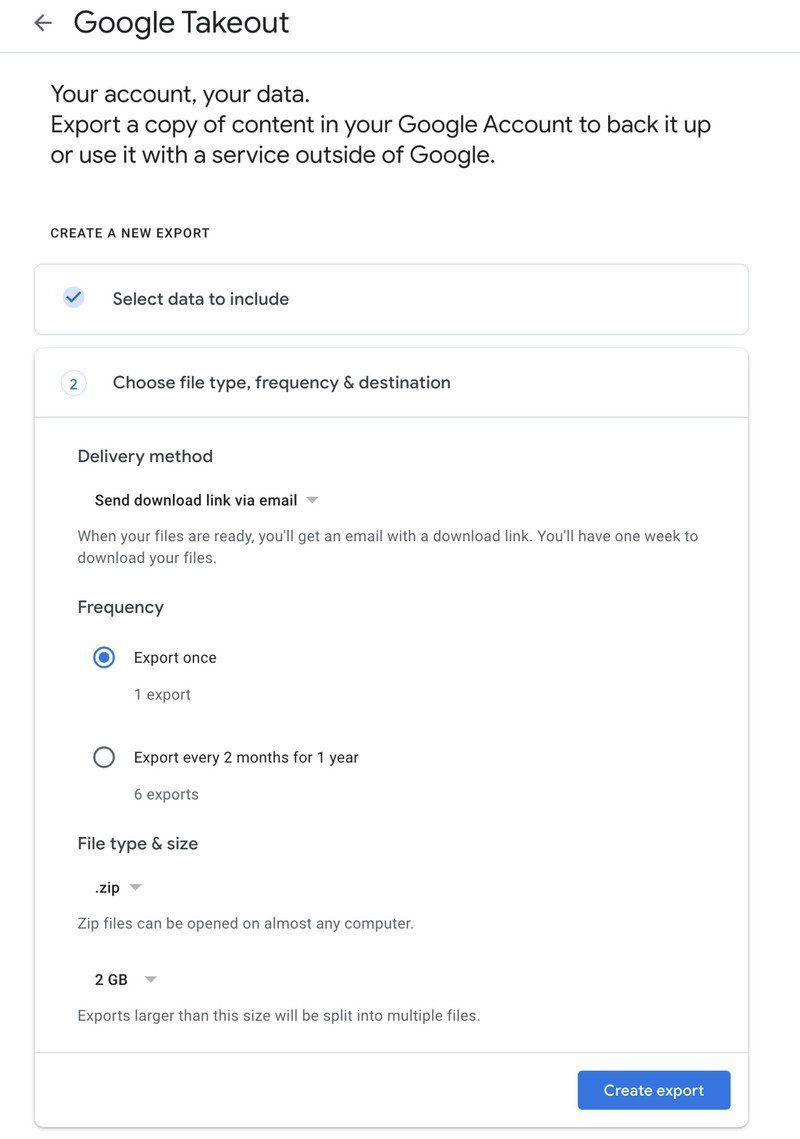The image pertains to Google Takeout, a service for exporting a copy of your Google account's data. At the top, there's a heading that reads "Google Takeout" accompanied by an arrow pointing left and the text: "Your account, your data. Export a copy of content in your Google account to back it up or use it with a service outside of Google."

Below this heading, a section labeled "Create a new export" appears. Within this section, a checkbox next to the text "Select data to include" is visible. Further down, there's another instruction to "Choose file type, frequency, and destination."

Next, the method of delivery is outlined, with a selected option indicating "Send download link via email." The instruction specifies that once the files are ready, an email with the download link will be sent to you, and you'll have one week to download your files.

Different options are presented under the "Frequency" section. The first option, labeled "Export once," has a blue dot indicating it is selected, whereas the second option is "Export every two months for one year" (six exports), and this one is unselected with an empty circle.

Under the "File type & size" section, the file format ".zip" is the default option with an explanation that zip files can be opened on nearly any computer. Additionally, it states that files larger than 2 GB will be split into multiple files. Finally, in the bottom right corner, there's a blue button labeled "Create export."

This detailed guide visually outlines the steps and options available to export data from your Google account using Google Takeout.